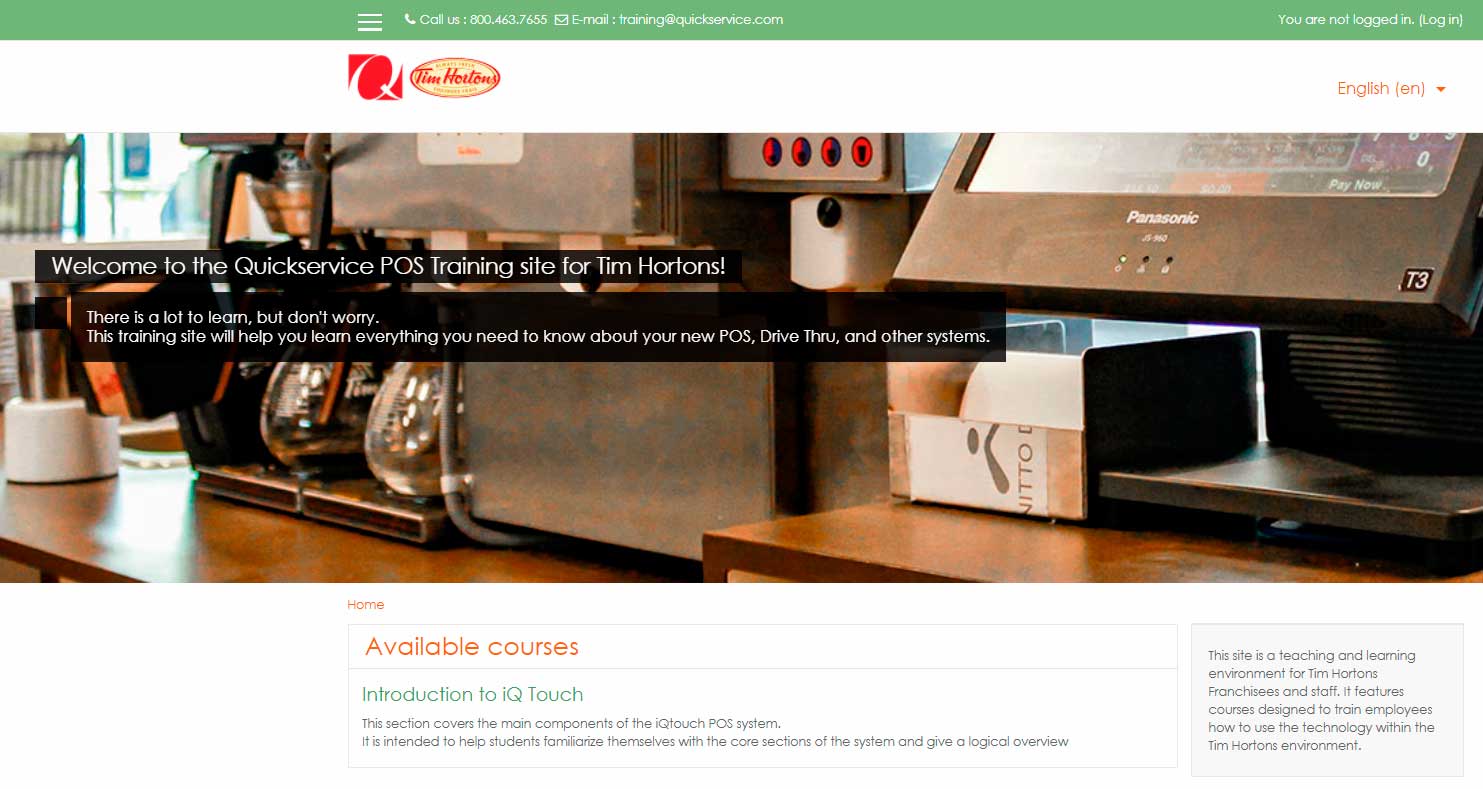The image is a screenshot from the Tim Hortons website, specifically a training page for their point-of-sale (POS) systems. At the top of the page, there is a green bar that includes an 800 number and an email address, both of which are too small to be read clearly. In the upper right corner, the page indicates "You are not logged in" with an option to log in.

Below the contact information, the Tim Hortons logo is prominently displayed. Adjacent to the login section, there is a language selection menu currently set to English, indicated by a drop-down arrow.

Central to the image is a large picture of coffee machines accompanied by a welcoming message. The text overlay reads: "Welcome to the Quick Service POS Training site for Tim Hortons. There's a lot to learn but don't worry. This training site will help you learn everything you need to know about your new POS, drive-through, and other systems."

Beneath this main section is a small button labeled "Home." Below the button, the heading "Available Courses" appears with a subheading "Introduction to IQtouch," followed by additional text that is too small to read clearly.

To the right of this course introduction, there is a description emphasizing that the site serves as a teaching and learning environment for Tim Hortons franchises and staff. It highlights that the website features courses designed to train employees on the technology used within the Tim Hortons ecosystem. The text in this section is light and small, making it difficult to read clearly.